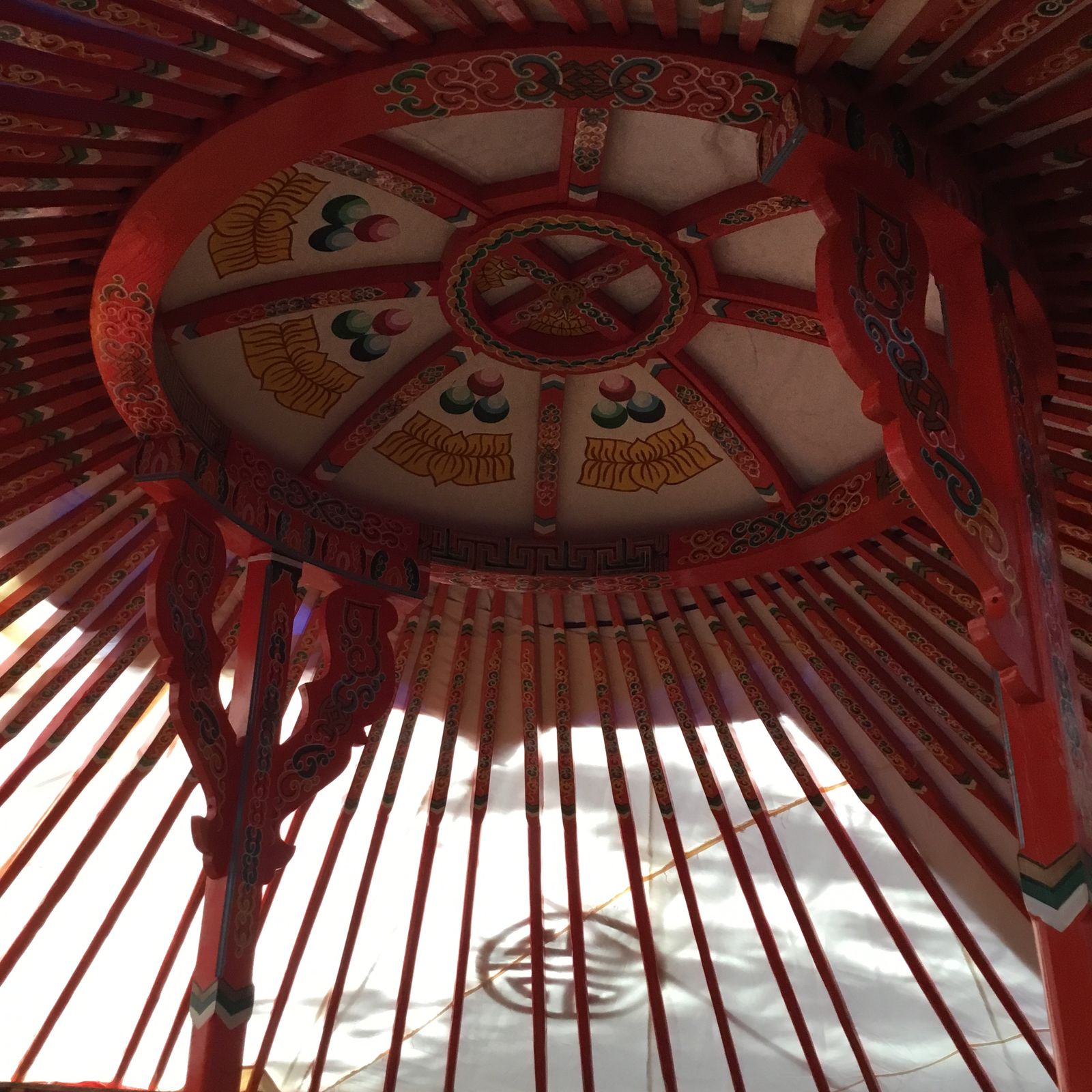This image captures the interior of a tent-like structure with a distinct circular, wheel-like design on the roof. The roof features an intricate pattern decorated in red, green, and white colors. The wheel-like design is adorned with red and blue balloon motifs and is reminiscent of an old-fashioned carnival wheel with spokes, although it appears stationary. The structure's walls are created using vertical bamboo poles, painted red with additional designs, spaced apart enough to reveal glimpses of the outside. Through these gaps, the sky is visible, accentuated by dark clouds, adding a dramatic contrast to the vibrant interior.